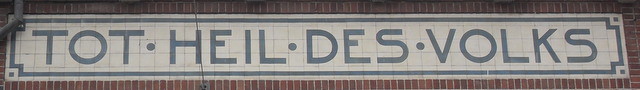The sign presented in the image features a series of words in another language, prominently displayed in capital letters. The text reads "T-A-U-T.", "H-E-I-L.", "D-E-S.", and "V-O-L-K-S.", with each of the four words separated by a dot. The background of the sign mimics a graph paper design, complete with small squares, and is painted in a grayish color. The sign is crafted from either metal or wood. The lettering and the border surrounding the text are both rendered in a grayish-blue hue, giving the overall presentation a consistent color scheme.